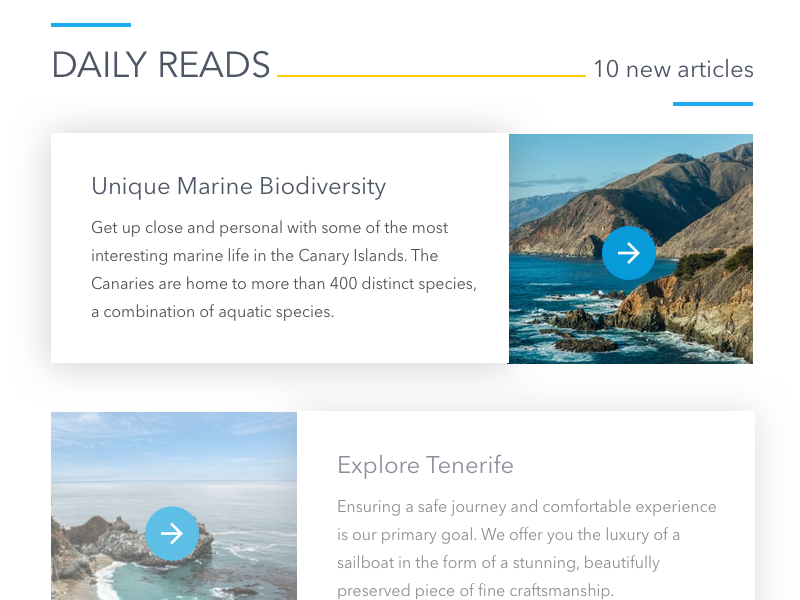**Caption:**

At the top of the page, the phrase "Daily Reads" is prominently displayed, highlighted by a blue line above and an orange line that extends to the right, leading to "Ten New Articles" in the top right corner, underlined in blue for emphasis.

Below this section, a wide box spans the width of the page with the headline "Unique Marine Biodiversity." This section invites readers to "Get up close and personal with some of the most interesting marine life in the Canary Islands," which are home to over 400 distinct aquatic species. 

Adjacent to this text is a stunning image of gently rolling mountains with waves crashing against the rocks below. An arrow appears in the center of the picture, directing users to explore further, and underneath, the text "Explore Tenerife" is featured in a grayed-out font, indicating an inactive dialog box.

Continuing down the page, another photograph showcases a similar rocky outcrop extending into calmer waters, under mostly blue skies with a few wispy white clouds. Text below highlights the enjoyment of a "safe journey and comfortable experience," offered through the luxury of a sub in a "sunny, beautifully preserved piece of fine craftsmanship."